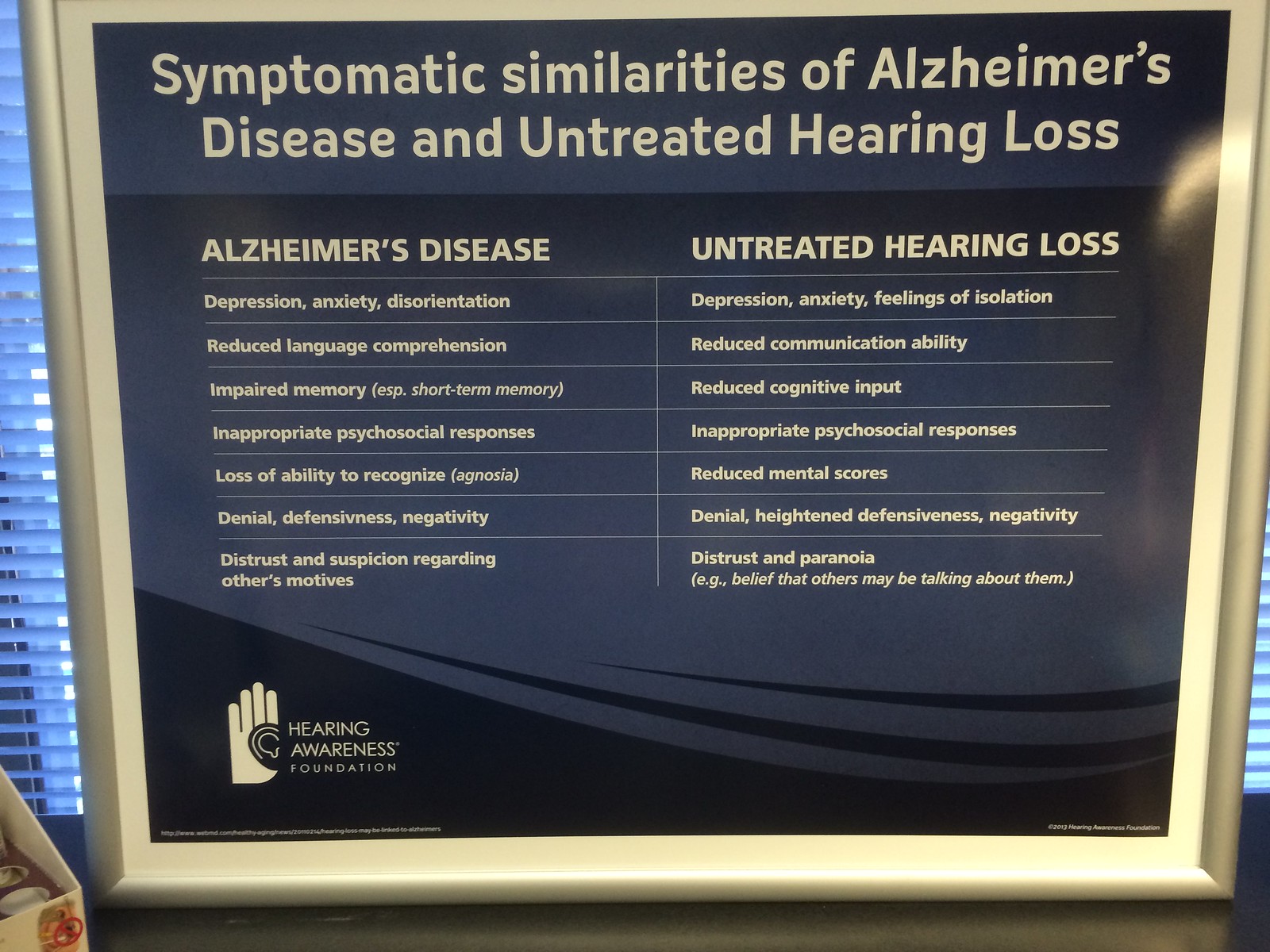The image features an informative signboard, likely situated in a healthcare setting, with windows and screens visible in the background. The central framed poster is displayed on a black platform with additional items present. The frame itself has a golden cream border with an internal light yellow border, against a backdrop of black and dark blue patterns and designs.

The poster's headline reads, "Symptomatic Similarities of Alzheimer's Disease and Untreated Hearing Loss." Below the title, the content is divided into two columns: the first column lists symptoms associated with Alzheimer's disease, including depression, anxiety, disorientation, reduced language comprehension, impaired memory (particularly short-term), inappropriate psychosocial responses, loss of ability to recognize (agnosia), denial, defensiveness, negativity, distrust, and suspicion regarding others' motives. The second column lists symptoms of untreated hearing loss, including depression, anxiety, feelings of isolation, reduced communication ability, reduced cognitive input, inappropriate psychosocial responses, reduced mental scores, denial, heightened defensiveness, negativity, distrust, and paranoia, such as the belief that others might be talking about them.

In the bottom left-hand corner of the poster, there's a logo featuring a hand holding an ear, symbolizing the Hearing Awareness Foundation, accompanied by the foundation's name. There is also a partially visible website footnote and in the bottom right corner, a copyright notice indicating the year 2013 and the Hearing Awareness Foundation.